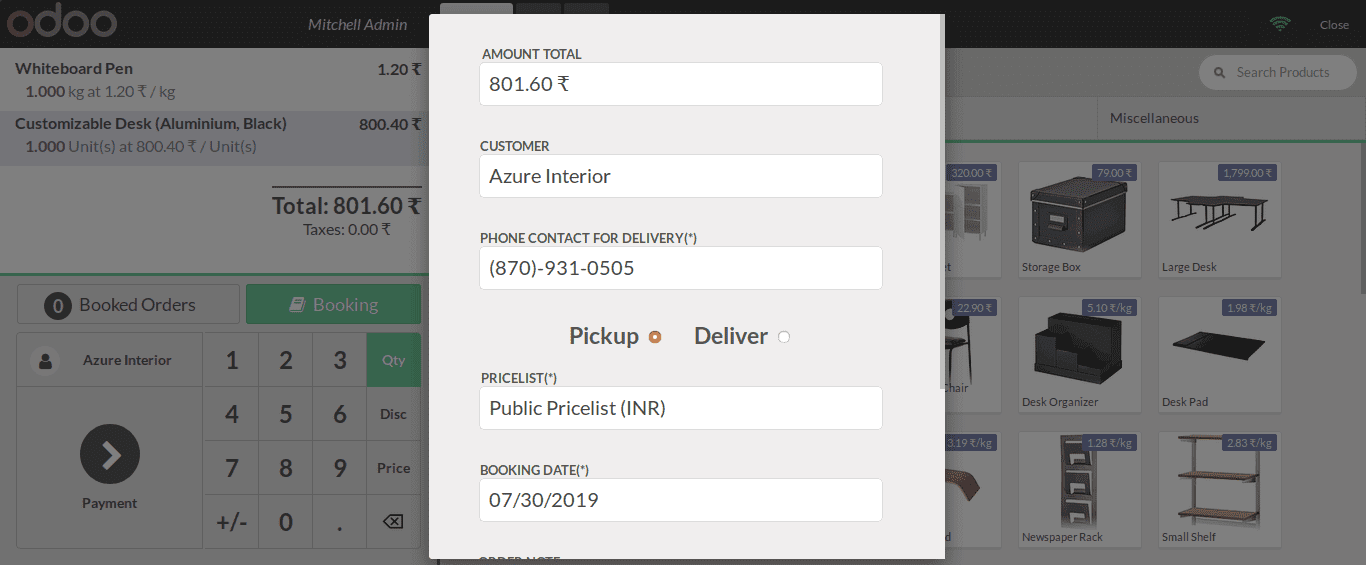In this image, the background reveals a cluttered workspace with several items and details outlined in a handwritten manner on a whiteboard. Among the written content, a photo of a whiteboard is seen along with a whiteboard pen. Numerical details are provided regarding the cost of certain items: for instance, 1 kilogram of arts (art supplies) is priced at 1.2 rupees per kilogram.

Additionally, there’s mention of a customizable aluminum desk with a black finish priced at 800.4 rupees per unit; 1 unit is listed, making the total cost 801.6 rupees. Notably, taxes stand at 0.00 rupees. The listed items include books, suggesting orders or bookings.

Details about the interior, specifically an "azure interior," are mentioned twice related to customer specifics and the payment process. A contact number (870-931-0505) is provided, presumably for delivery purposes, while "pickup" is also an option. The public price list is indicated to be in Indian rupees, with a booking date noted as July 30, 2019.